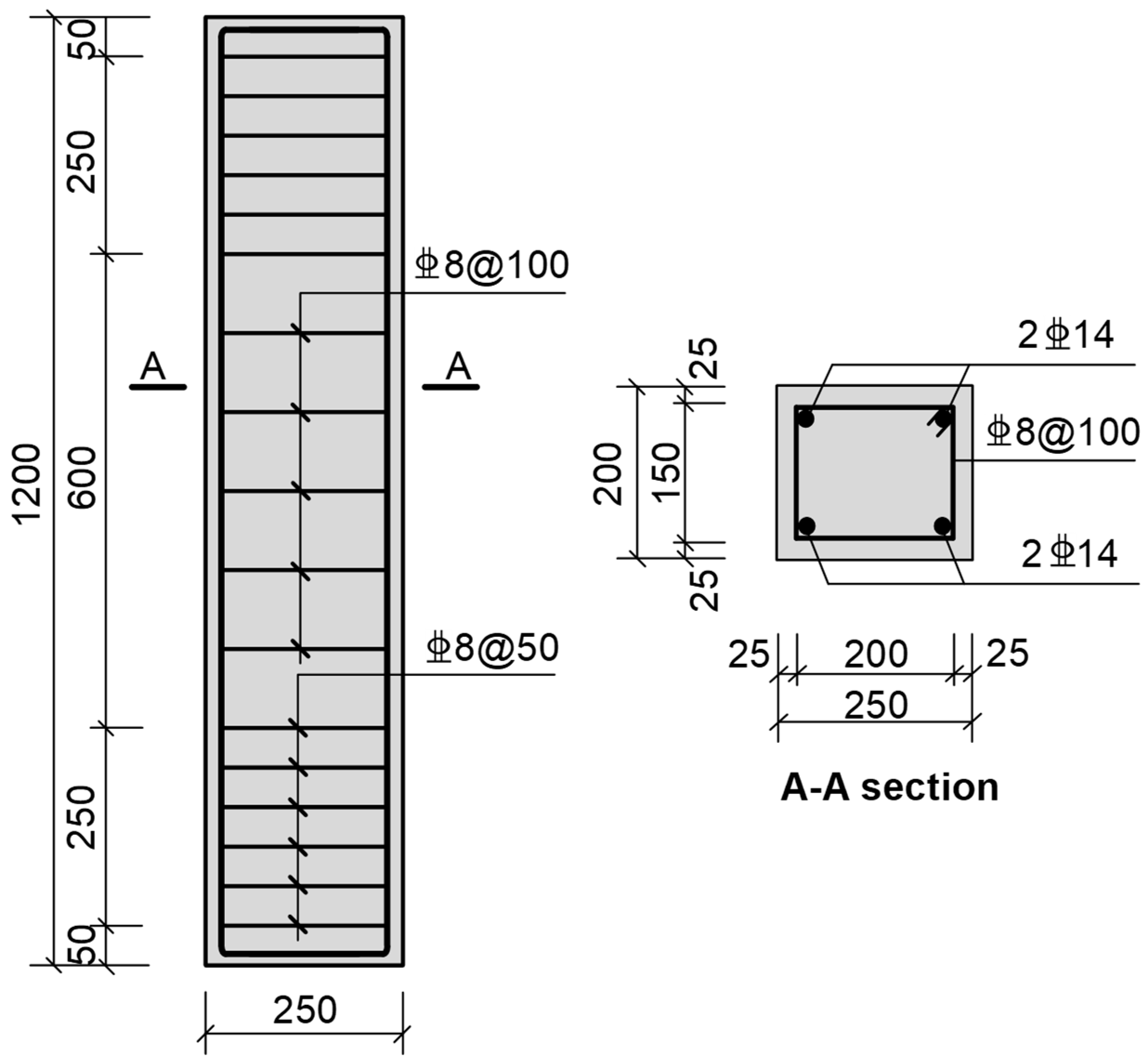The image is a square print featuring a light gray and black two-tone color scheme, set against a solid white background. On the left side, there is a vertically oriented gray rectangle divided into segments by black lines, with numbers along the left edge: 1200, 50, 250, 600, 250, and 50. Inside the rectangle, there are various numbers, such as 8, 100, and 8, 50. To the right of this, there is an additional section of text featuring numbers like 214, 8 at 100, 214, 200, and 250. A blue square sits at the center-right of the image, containing more numbers and symbols. Additional details include black borders inside the gray rectangle and black bolded text at the bottom reading "AA section." The numbers and symbols scattered throughout the image contribute to its complex and structured appearance, although their meanings remain unclear.